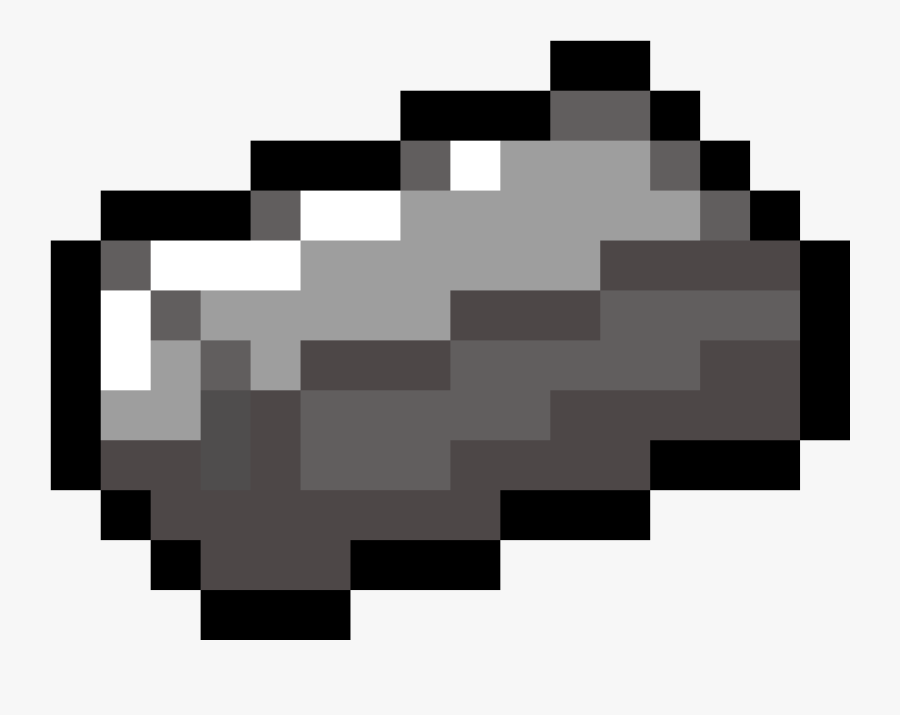This image features a single, centrally positioned object, clearly a low-resolution, digitally created item reminiscent of older video games, particularly those from the 90s or pixel art styles. The background is a solid plain white, providing a stark contrast that highlights the item. The object itself is a pixelated depiction of what appears to be an iron ore, characterized by its blocky structure and various shades of gray: light gray, dark gray, and black, with some parts accented by white to suggest a shinier surface. The item has a distinct black-lined border, giving it a defined, almost three-dimensional appearance. The grayscale colors are distributed in a diagonal pattern, with darker tones at the bottom transitioning to lighter grays and whites towards the top. The overall aesthetic, with its simplistic and nostalgic design, is highly evocative of games like Minecraft, where players would smelt ores to obtain iron bars.